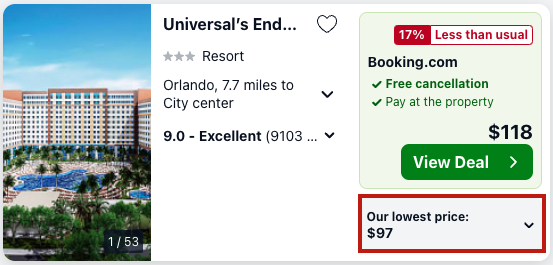This image showcases a snapshot from the travel website Booking.com, specifically highlighting a resort in Orlando. On the far left, the picture prominently displays the resort itself, a tall and expansive building featuring multiple floors with numerous rooms aligned symmetrically on the left, right, and center. Beneath the towering structure, we notice a lush area adorned with trees encircling a sparkling pool.

In the bottom right corner of the image, a notation indicates that this is image 1 of 53, providing an option to swipe through additional images of the resort. Adjacent to the image, a white box contains the resort's name, "Universal's End," accompanied by a heart symbol for favoriting the listing and a three-star rating. 

The resort is located in Orlando, approximately 7.7 miles from the city center, a detail clearly highlighted for potential travelers. Additionally, the resort holds an impressive rating of 9.0, categorized as "Excellent." Further details to the right reveal a promotional discount, indicating that the current price is 17% less than usual. Booking.com offers free cancellation policies and the option to pay at the property, with prices highlighted at $118 and a special deal at $97, emphasizing their lowest price guarantee.